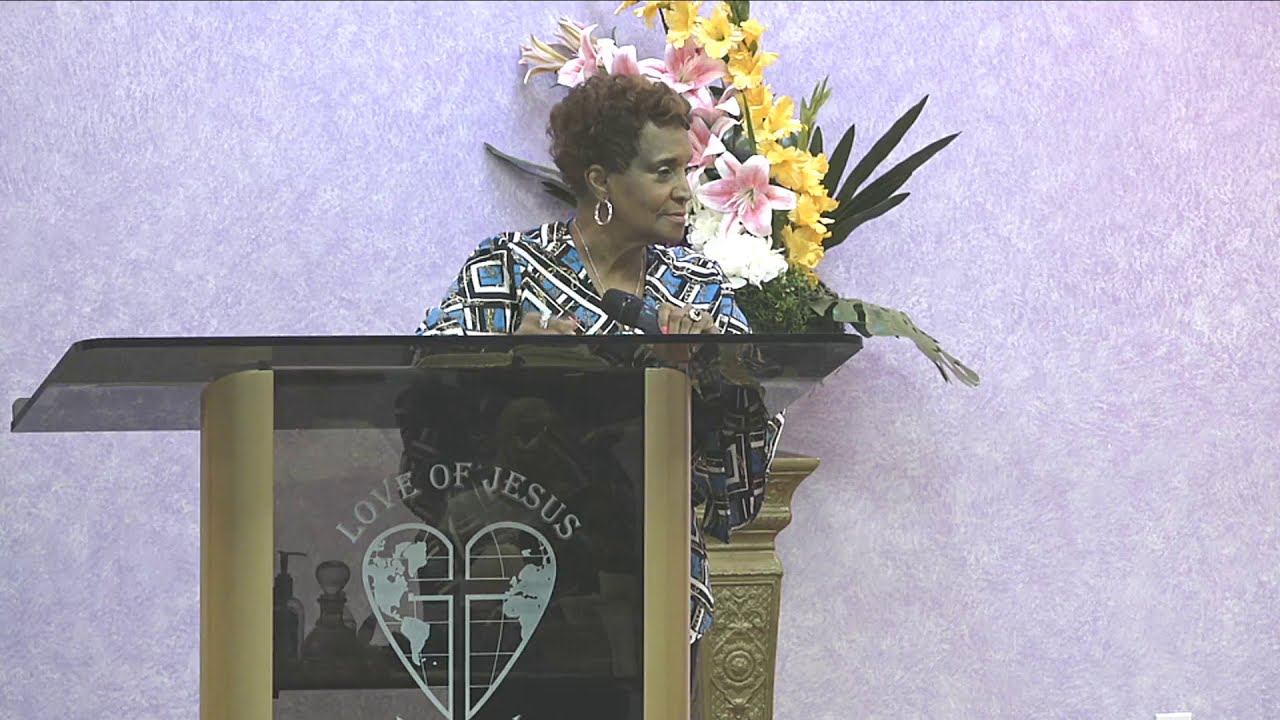In the image, an African-American woman with short black hair, adorned with hoop earrings, a necklace, and rings, is standing at a large, ornate podium, likely within a church setting. The podium is a striking black glass with bronze-colored sides and features a prominent etching on the front that reads, "Love of Jesus." Below the inscription, a heart-shaped globe with a cross at its center is intricately designed. The woman is holding a microphone in her left hand, resting it on the podium. She is dressed in a vibrant, long-sleeved top featuring blue, white, and black geometric patterns. Red lipstick adds a touch of boldness to her look. Behind her, set against a textured blue and light purple backdrop, there is a tall, narrow stand supporting a large flower arrangement with pink stargazer lilies, yellow and white blossoms, and green leaves, all in a gold vase. This elegant and spirited scene is captured in a detailed photograph.